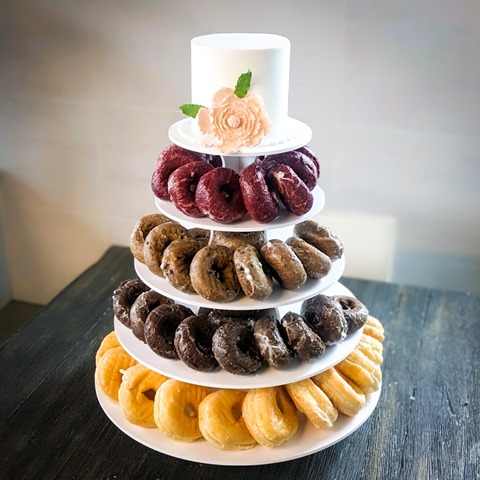This detailed, color photograph captures an indoor scene featuring a unique wedding cake crafted entirely from doughnuts, meticulously arranged on a tiered spinning stand. The doughnuts are placed on circular shelves that diminish in size as they ascend, forming a triangular or Christmas tree shape with four distinct layers. The entire setup rests on a large white plate on a table with a gray and tan surface, set against a light gray wall.

The bottom and widest tier is adorned with numerous plain cake vanilla glazed doughnuts, showcasing a light yellow color. Moving upwards, the second tier presents a selection of rich chocolate glazed doughnuts, slightly fewer in number. The third tier features blueberry glazed doughnuts, distinguished by their light brown hue, continuing the pattern of decreasing size and quantity. The top and smallest tier is adorned with dark red, red velvet cake doughnuts, completing the tiered structure.

At the pinnacle of this dessert tree is a decorative white cylinder crowned with a frosting rose in a peach hue, flanked by two green rose petals, adding an elegant finishing touch to the composition. The photograph's style of representational realism vividly captures the intricate details and textures of each doughnut and the overall visual arrangement, making it a striking and delectable focal point.